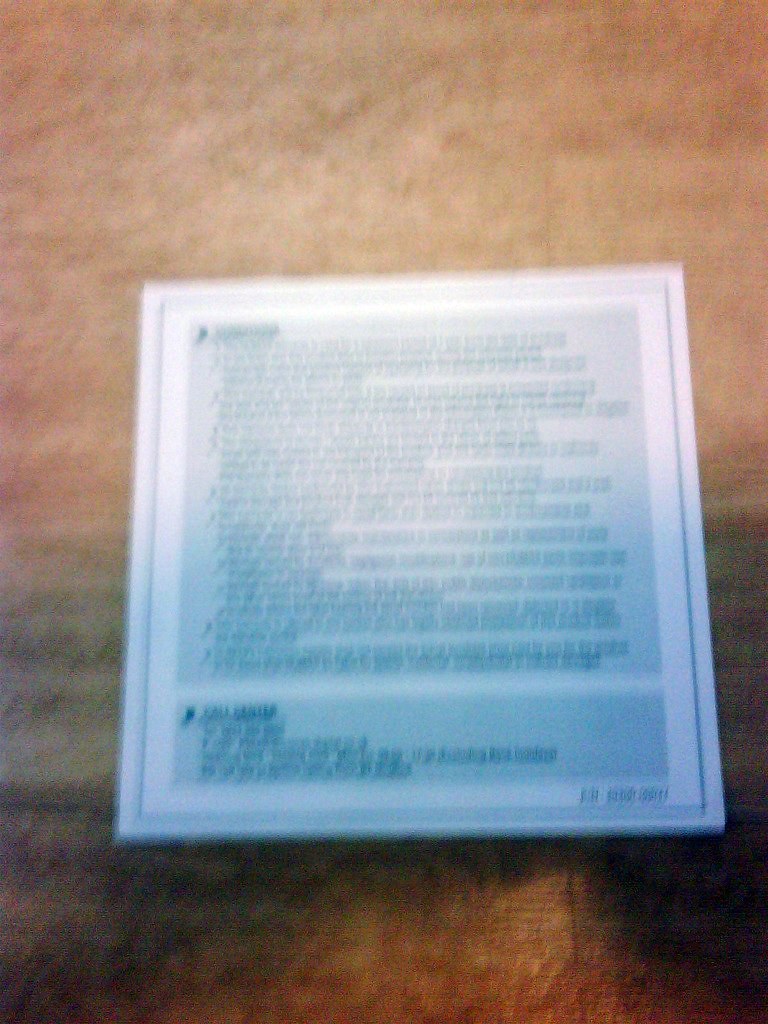The image depicts an extremely out-of-focus document, which initially appears to be lying on a table but upon closer examination seems to rest on a hairy surface, possibly someone's chest. The document features a blue border enclosing a white sheet of paper. Inside, printed text is arranged in a lighter blue section, divided into two parts: two paragraphs. The upper paragraph is notably longer—approximately five times the length of the shorter one at the bottom. Each section is headed by an underlined title accompanied by a small, indistinct bullet point. The blur makes the text and finer details practically unreadable.